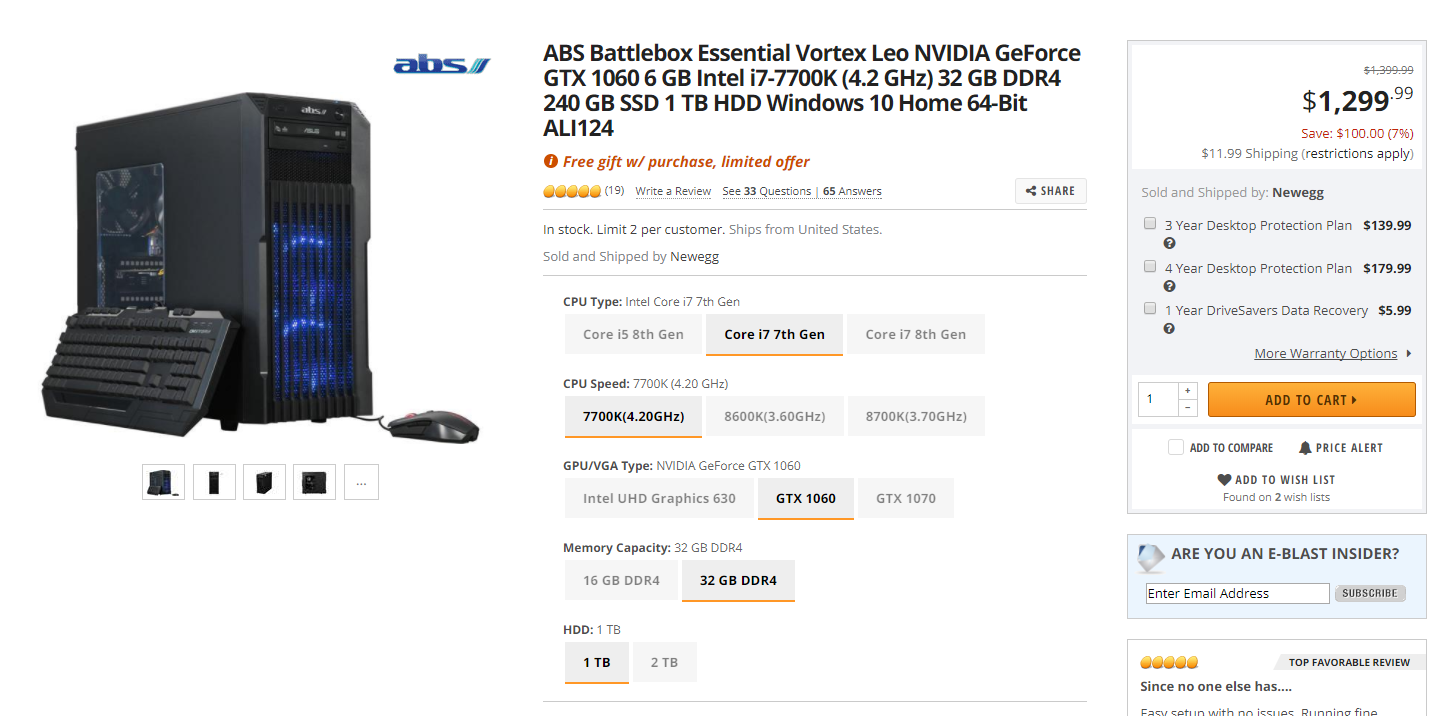This image showcases a black desktop computer, with an accompanying black keyboard leaning against it. A mouse is also present next to the setup. Below the main image, there are four thumbnails that offer alternative views of the same product. This image is sourced from the ABS website and features the ABS Battlebox Essential Vortex Leo, which comes with an NVIDIA GeForce GTX 1060 6GB graphics card and an Intel i7-7700K processor.

The product page allows buyers to customize several components, including the CPU type and speed (with three options available), the GPU/VGA type (also three options), memory capacity (choose between 16GB or 32GB), and HDD storage (either 1TB or 2TB). The current price of the desktop is listed at $1,299.99, with an orange button to add the product to the cart situated on the right side of the screen.